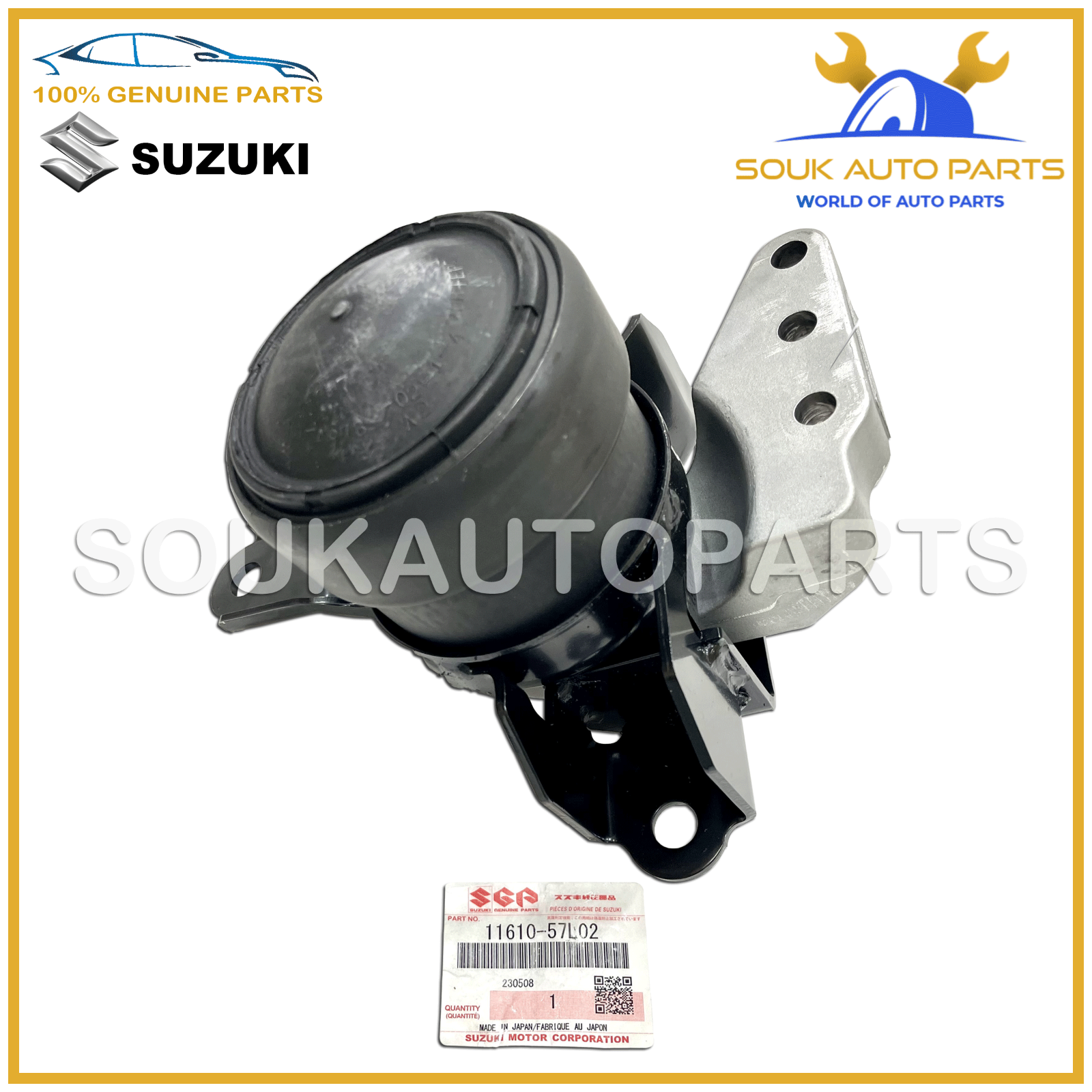This detailed image of an automobile part, likely intended for an online listing rather than a catalog, prominently features several distinctive elements confirming its authenticity and source. At the top of the photograph, the caption "100% Genuine Parts" is accompanied by the "Suzuki" logo. In the upper left corner, a blue outline of an automobile reinforces the Suzuki branding. The upper right corner displays a blue tire with two gold wrenches emerging from it, alongside the text "Souk Auto Parts, World of Auto Parts" in blue and gold lettering.

The primary object in the center is a metallic auto part, likely a starter motor, featuring a combination of gray and silver components with some black housing. It has multiple brackets: one on the right with three drilled holes for bolts, and additional brackets below and to the left, each with a drilled hole for mounting purposes. Below the auto part, a Suzuki Motor Corporation tag is visible, complete with a UPC and QR code, providing further evidence of the part's authenticity. A gold border frames the entire image, adding a final touch of credibility and detail to the presentation.